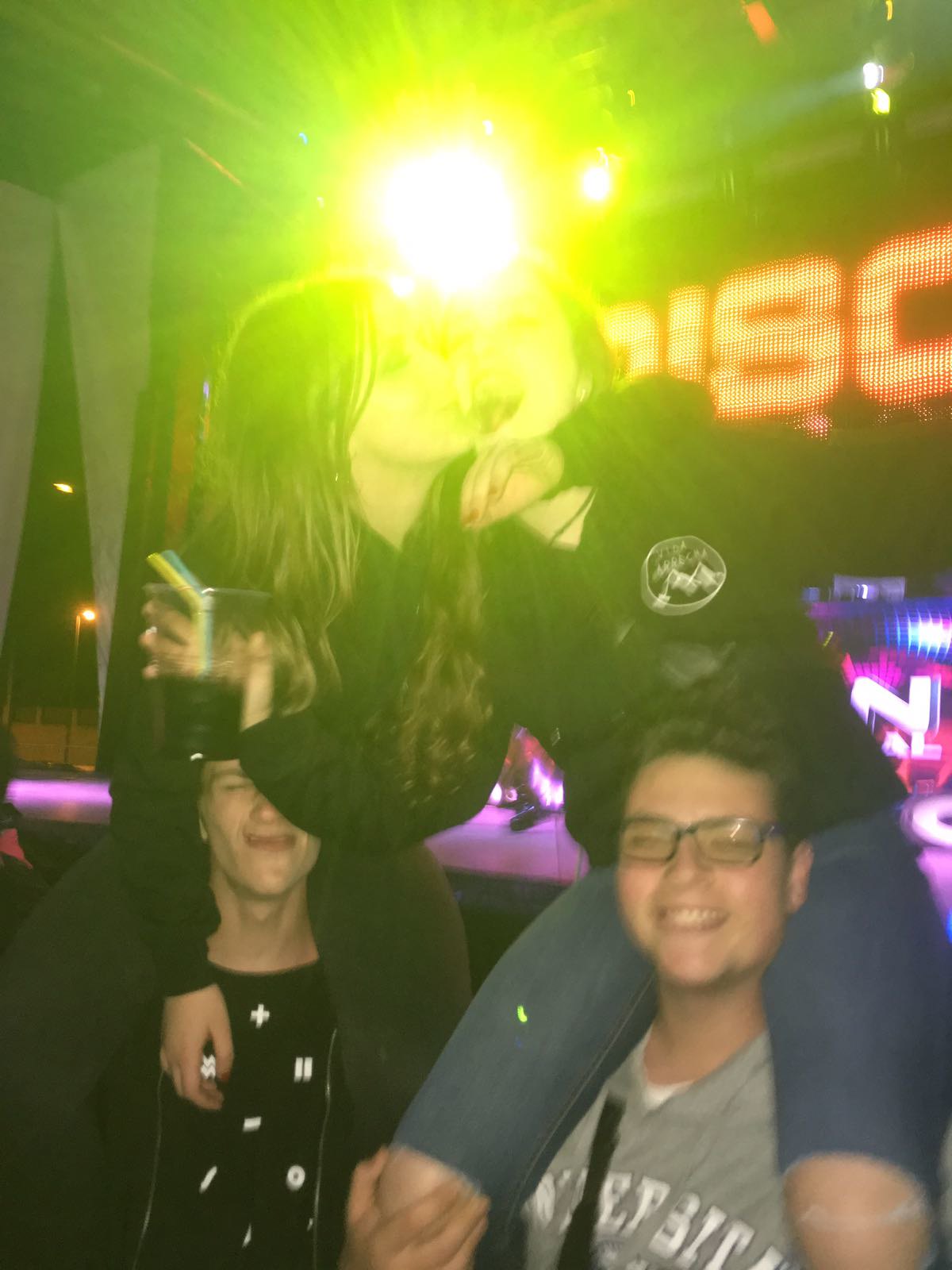In this vibrant and dynamic photo taken at a concert, a group of four friends—two boys and two girls—celebrates energetically in front of a brightly lit stage. Both boys, one in a black tank top with small white logos and the other in a gray t-shirt with a school's name in white letters, are hoisting the girls onto their shoulders. The girl on the right, dressed in a black shirt and jeans with holes at the knees, holds a clear cup with a dark drink and two straws. Her face is obscured by a powerful yellow stage light that also makes the entire scene appear slightly blurry. On the left, the other girl, clad in all black, has her legs wrapped around the boy’s shoulders and is kissing or hugging her friend. Behind them, the stage, adorned with purple lighting and possibly reading "disco" in orange letters, adds to the concert’s lively atmosphere. Their shared joy and the concert’s energy are palpable despite the blurriness from the stage light.